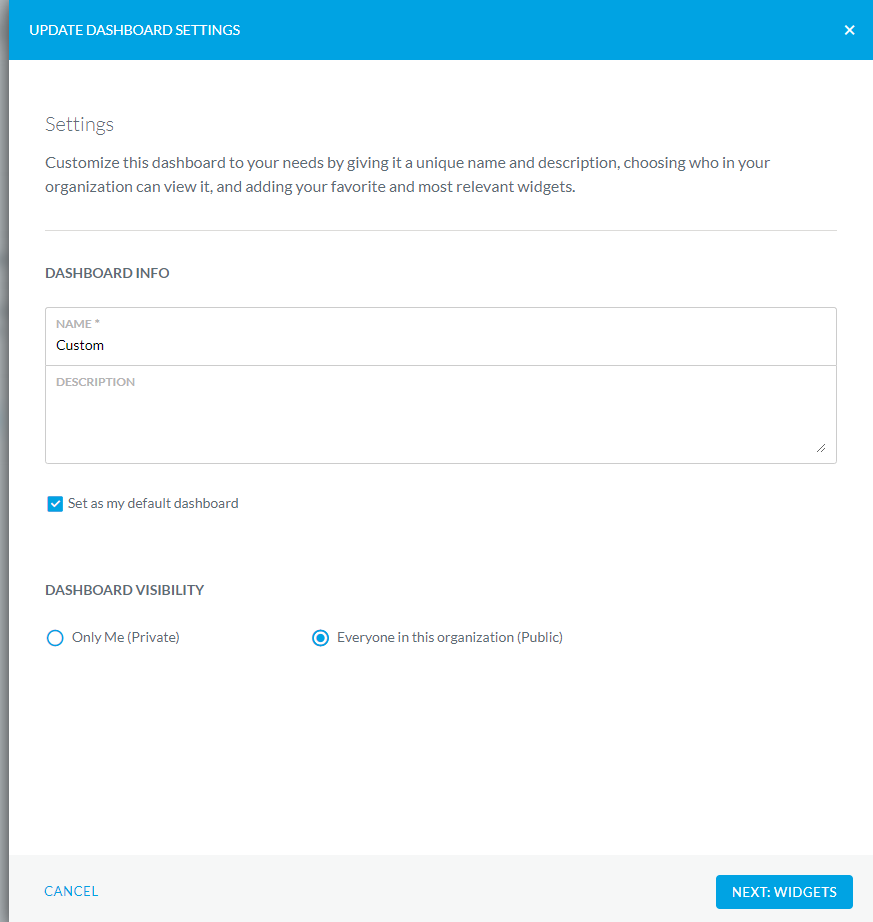The image depicts a screenshot captured from a desktop computer screen, specifically showing a window from an application. The window features a white background with a blue horizontal bar at the top. On this blue bar, white capital letters state "UPDATE DASHBOARD SETTINGS." Positioned in the upper left corner of the screen, this title clearly indicates the purpose of the window.

In the main body of the window, the background remains white and a detailed text description is provided. The text reads: "Settings. Customize this dashboard to your needs by giving it a unique name and description, choosing who in your organization can view it, and adding your favorite and most relevant widgets." This text is underlined by a faint gray line, distinguishing it from the subsequent sections.

Below this introductory text, the section titled "Dashboard Info" is visible. It includes a form that consists of several radio buttons and various controls, enabling users to input or select data according to their preferences. Finally, at the bottom of the page, aligned to the lower right, there is a prominent blue button with white text that reads "NEXT: WIDGETS." This button likely serves as a navigation tool to continue the dashboard customization process.